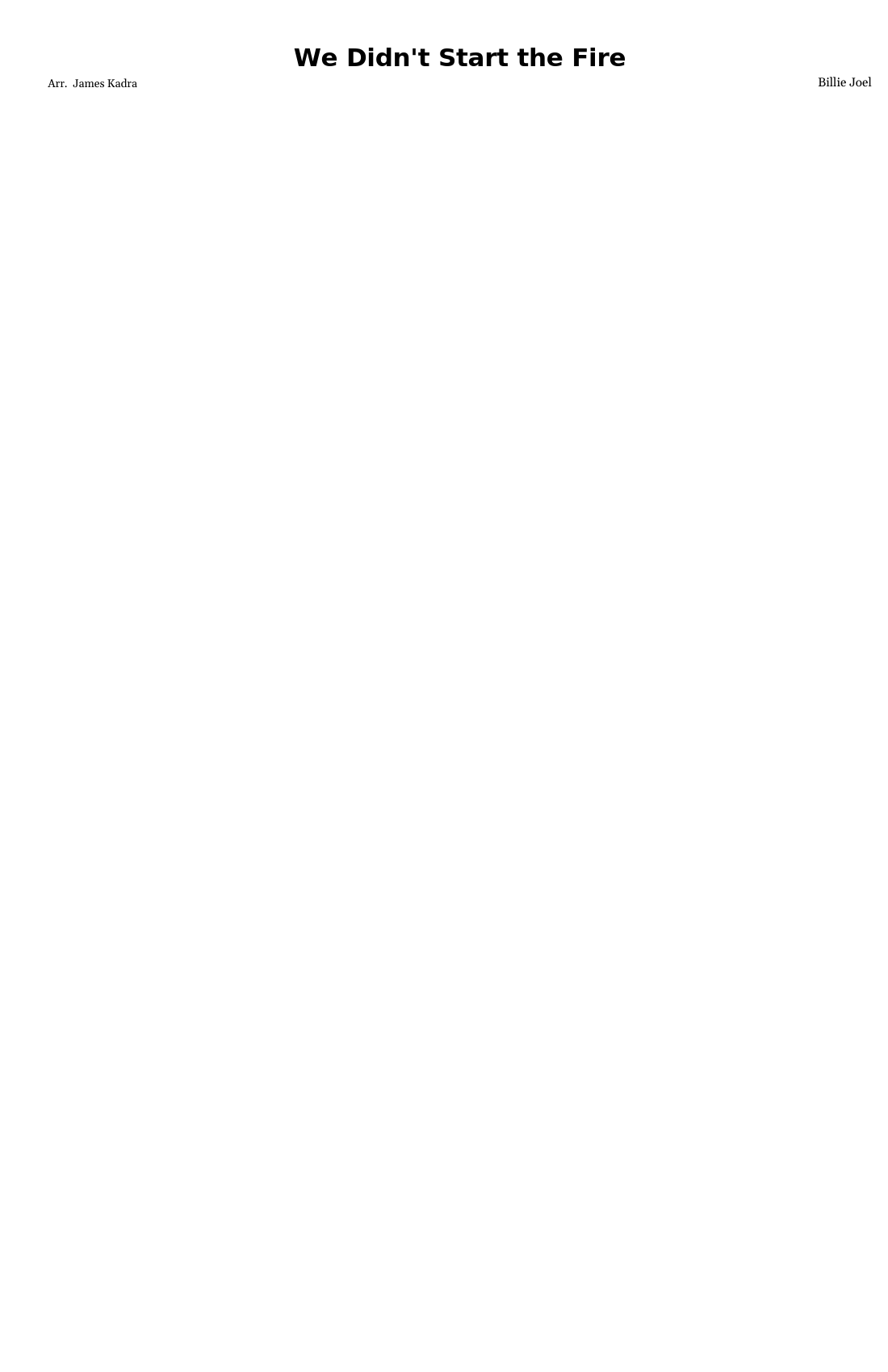The image depicts a nearly blank sheet of paper, seemingly intended for writing or typing the lyrics to Billy Joel's song "We Didn't Start the Fire." Only three distinct segments of text are present on the otherwise empty page:

1. **Upper Left Corner**: The text "ARR. JAMES KADRA" is noted, possibly indicating the arranger or another associated individual.
2. **Upper Right Corner**: The name "Billy Joel" is prominently displayed, acknowledging the creator of the song.
3. **Center of the Page**: In a larger, bold font, the title "We Didn't Start the Fire" is clearly marked, emphasizing the song's title.

The rest of the paper remains blank, suggesting that the transcription of the lyrics was either unfinished or encountered some typographical issue that resulted in the majority of the text not being displayed. This incomplete document hints at an interruption or an error occurring during the preparation.